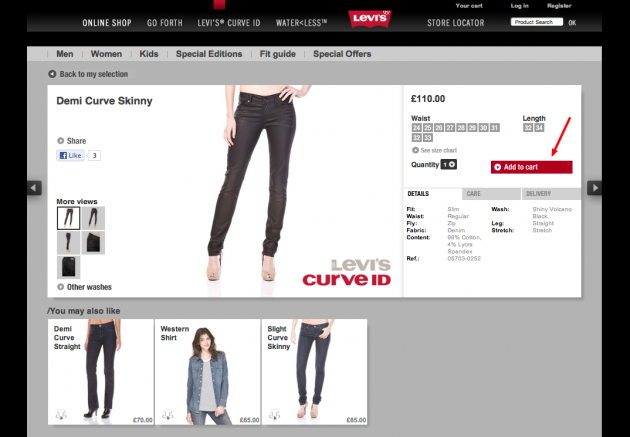The image is a screenshot from the Levi's website. The background is predominantly black, with a gradient black navigation bar at the top. The navigation bar features white text, listing options such as "Online Shop," "Go Forth," "Levi's Curved ID," "Waterless," and the iconic red Levi's logo. Additional options include "Store Locator" and a search bar.

Below the navigation bar is a catalog showcasing various jeans, divided by styles such as "Curved ID" and "Skinny," with prices listed at 110 euros or pounds. The catalog includes a range of jeans and a jean jacket, available for both tall and short individuals. Each product listing provides options to select waist size and length, with some sizes shown in light gray to indicate limited availability. Users can also navigate to sections titled "Care" and "Delivery."

Models in the catalog images are pictured wearing high heels with their jeans. The page continues with a gray background below the main catalog section, maintaining a sleek and modern aesthetic throughout the site.